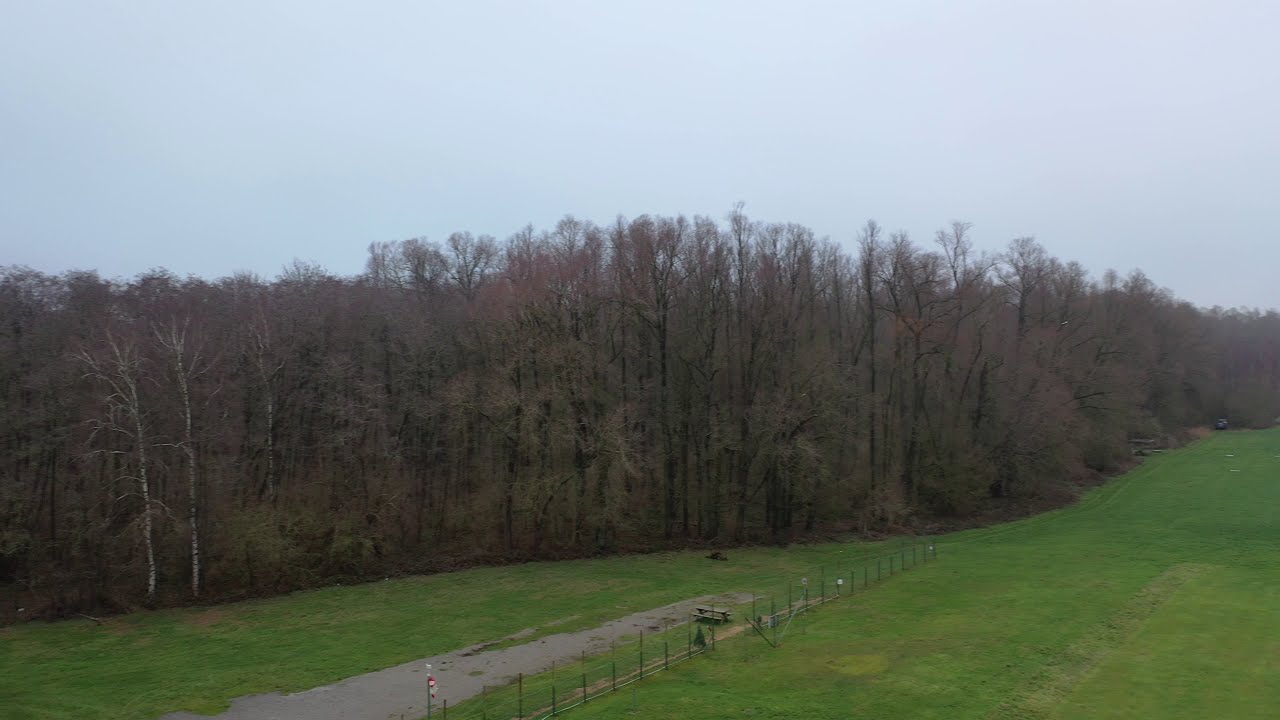This photograph, taken on a cloudy day, captures a large, recently mowed grassy field with visible lawnmower treads. A small, thin fence runs diagonally from the center right to the bottom center of the image, delineating the field. To the left of the fence, there is a walked path cut into the grass, and further left, remains of a once-paved road now overgrown with grass. The field is bordered by a dense tree line of mostly barren trees, leading into a wooded area. Above the treeline, the dreary gray sky dominates, contributing to the overall atmospheric feel of the scene.